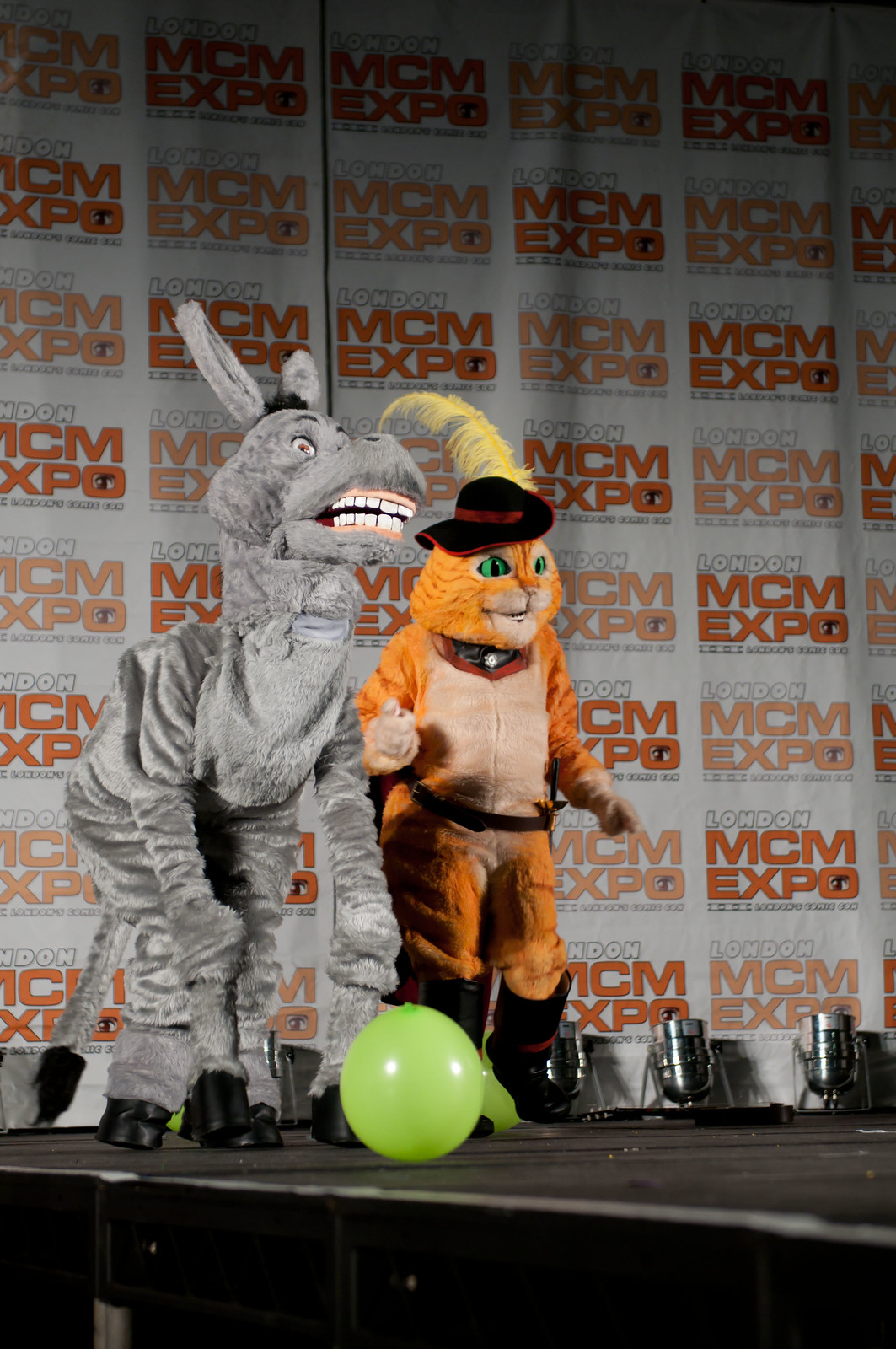In this detailed image, we see two individuals dressed as iconic fictional characters on a black stage. To the left, there's a person in a grey donkey suit with big teeth, likely portraying Donkey from "Shrek". The donkey has large white teeth, pink gums, and black hoofs. In front of him lies a green balloon. To the right, stands an orange tabby cat with big green eyes, identifiable as Puss in Boots, complete with his signature black hat adorned with a yellow feather, a red trim, and a pair of boots. Behind them, the backdrop features several logos with "London" written in white and "MCM Expo" in orange, suggesting the setting is a comic or pop culture convention. Also in the background are silver drums placed on the stage. This vivid scene captures the essence of a vibrant cosplay event.